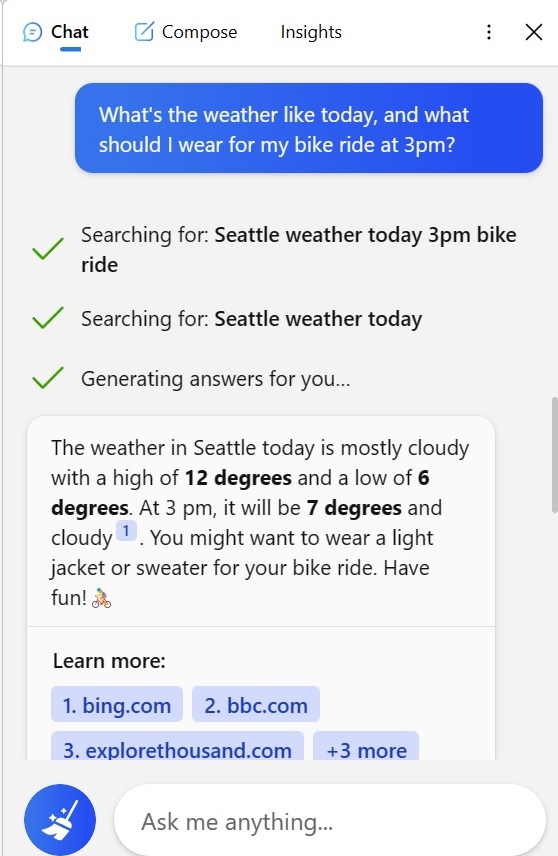The screen displays the results of a query within a multi-tab interface featuring the labels "Chat," "Compose," and "Insights" at the top, with "Chat" highlighted in blue. The user has asked, "What's the weather like today and what should I wear for my bike ride at 3pm?" The system is actively processing the query, indicated by the text, "Searching for Seattle weather today 3pm bike ride," accompanied by a green check mark signaling progress.

The response generated states, "The weather in Seattle today is mostly cloudy with a high of 12 degrees Celsius and a low of 6 degrees Celsius. At 3pm, it will be 7 degrees Celsius and cloudy." The text suggests, "You might want to wear a light jacket or sweater for your bike ride. Have fun." A "Learn more" link follows, along with two source references: "1. bing.com" and "2. bbc.com," indicating that the detailed weather information, specifically the 3pm forecast, was sourced from bing.com.